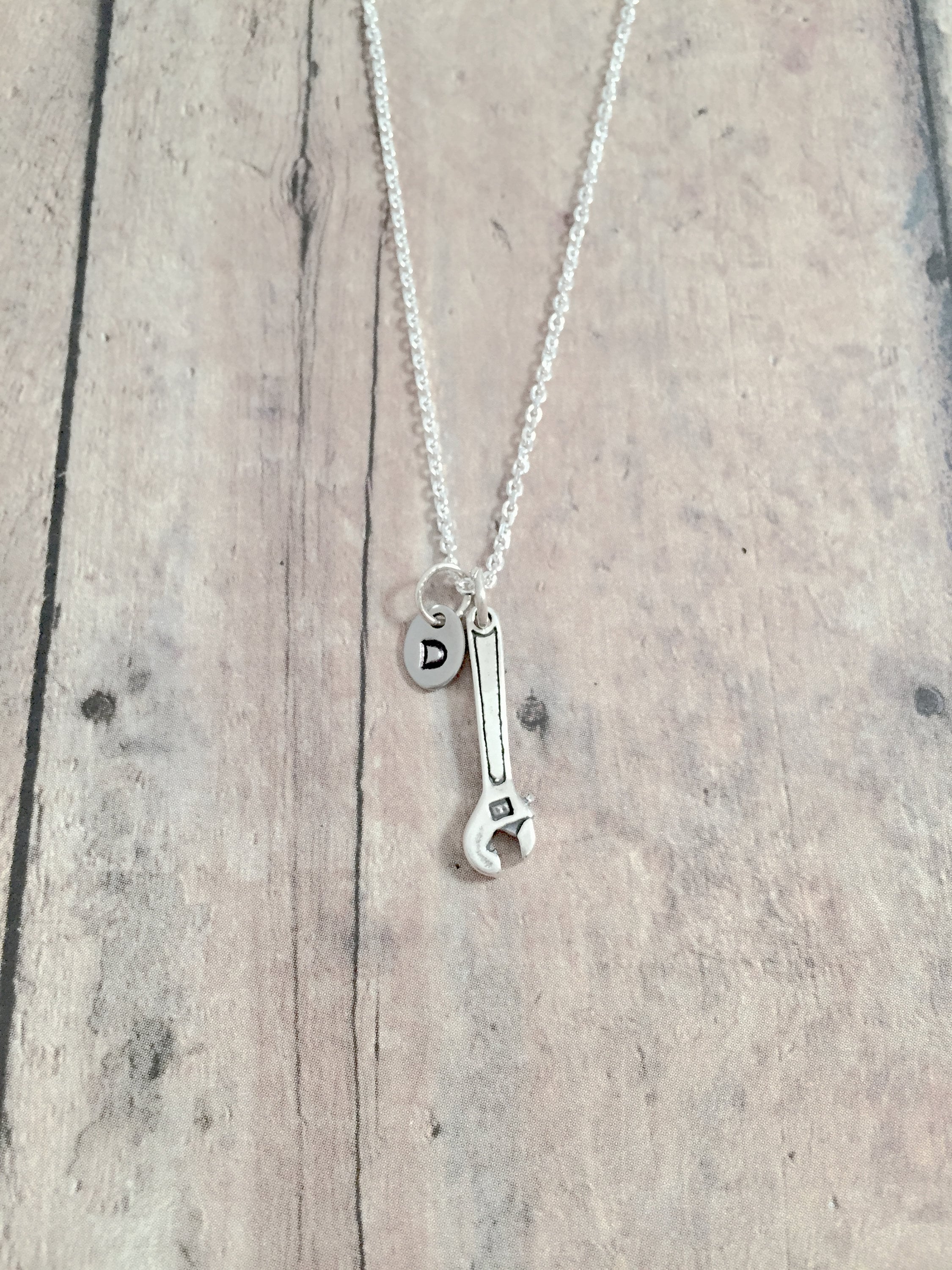The photograph showcases a silver necklace hanging on a rustic, light-colored wood surface, possibly a bleached or light white wood. The wood background, which has a rough, knotty texture typical of a rustic setting, might be part of a picnic table or similar outdoor furniture. The necklace itself features interlocking round chains, giving it a substantial and solid appearance. Dangling from the necklace is a small, intricately detailed crescent wrench charm, complete with an adjustable screw mechanism. Additionally, there is a metal disc charm inscribed with the letter "D." The necklace appears to be robust and hefty, suggesting it could be worn by someone for whom these charms hold significant personal meaning, possibly a mechanic or someone with an affinity for tools.